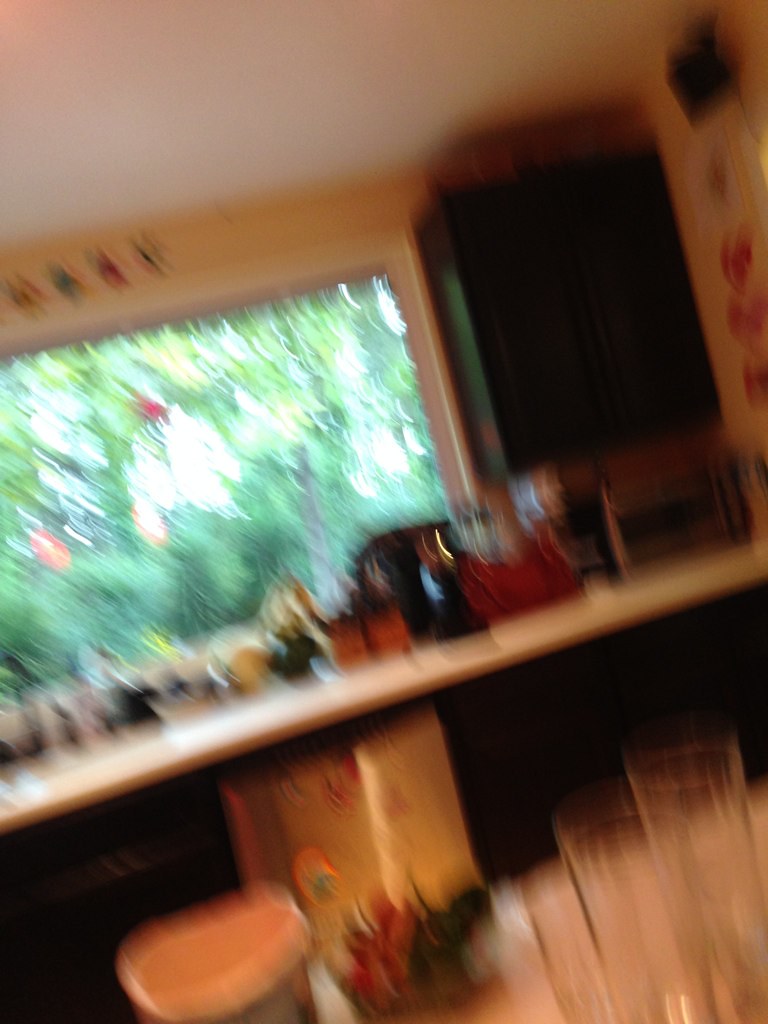This photo captures a slightly blurry room with a prominent white table at the center. The table hosts a couple of clear cups and a red and green arrangement, likely a plant or possibly strawberries. To the left of this are a white bowl and a brown box that appears to be under a counter. The white counter, cluttered with numerous indistinct objects in colors ranging from red, black, orange, yellow, white, blue, and green, is topped by a black cabinet on the wall in the top right corner. Below the cabinet sits a silver rectangle. The wall features some red decorations, while a large window offers a glimpse of greenery outside. Above the window are additional items in red, green, and yellow.